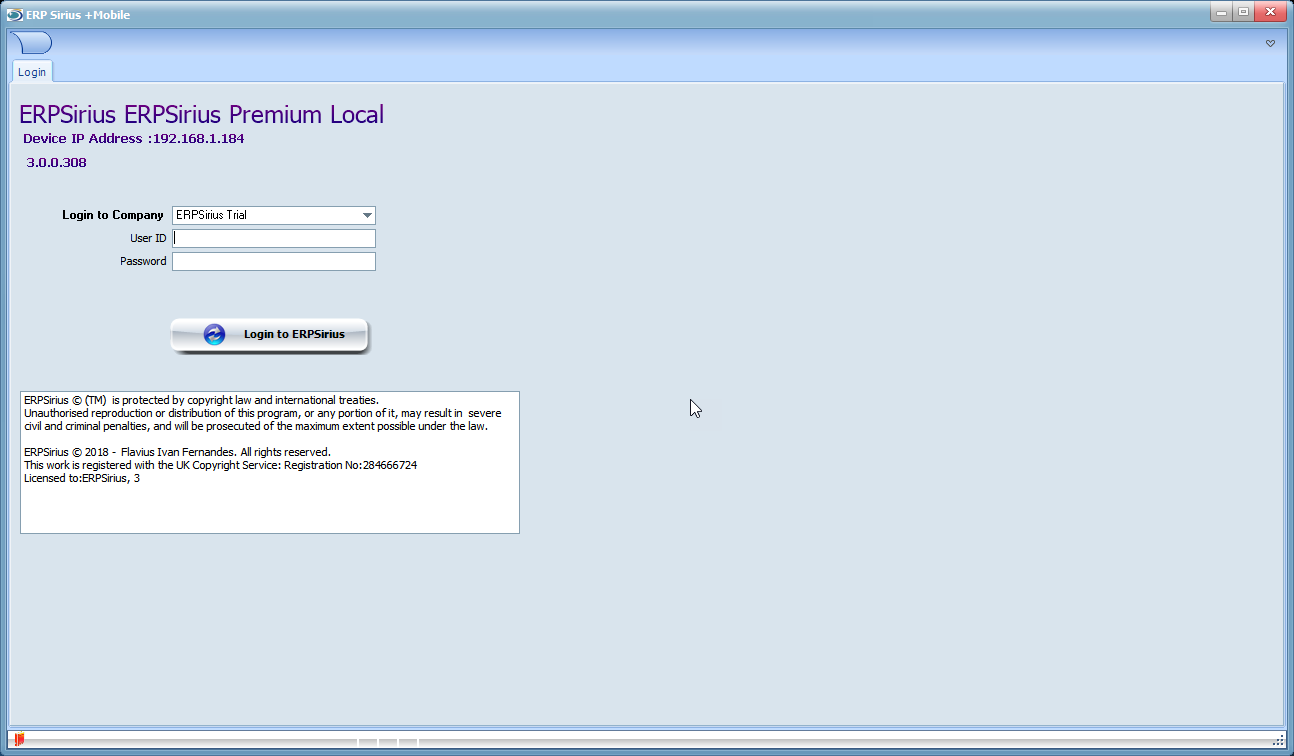The image depicts a web page for ERP Sirius, specifically the ERP Sirius Premium Local version. At the top, the page displays the title "ERP Sirius" followed by the version name. An IP address is also visible. The main section features a trial login interface, with separate input boxes for the user ID and password, accompanied by a prominent "Login" button.

Beneath the login interface, a detailed copyright notice is included, outlining the copyright owner's information, licensing details, and the copyright registration number. The notice is displayed on a white background.

The web page's header area is blue, while a light grey border appears at the bottom. The header in the top left corner reads "ERP Sirius Plus Mobile," indicating that this is likely a mobile-optimized page. The page includes typical window controls such as minimize, expand, and close, suggesting that the web page could simulate a desktop application interface as well.

Overall, the user interface elements, such as input boxes and the copyright snippet, are all white, enhancing readability. The design is clean and visually clear, focusing on a functional and straightforward user experience.